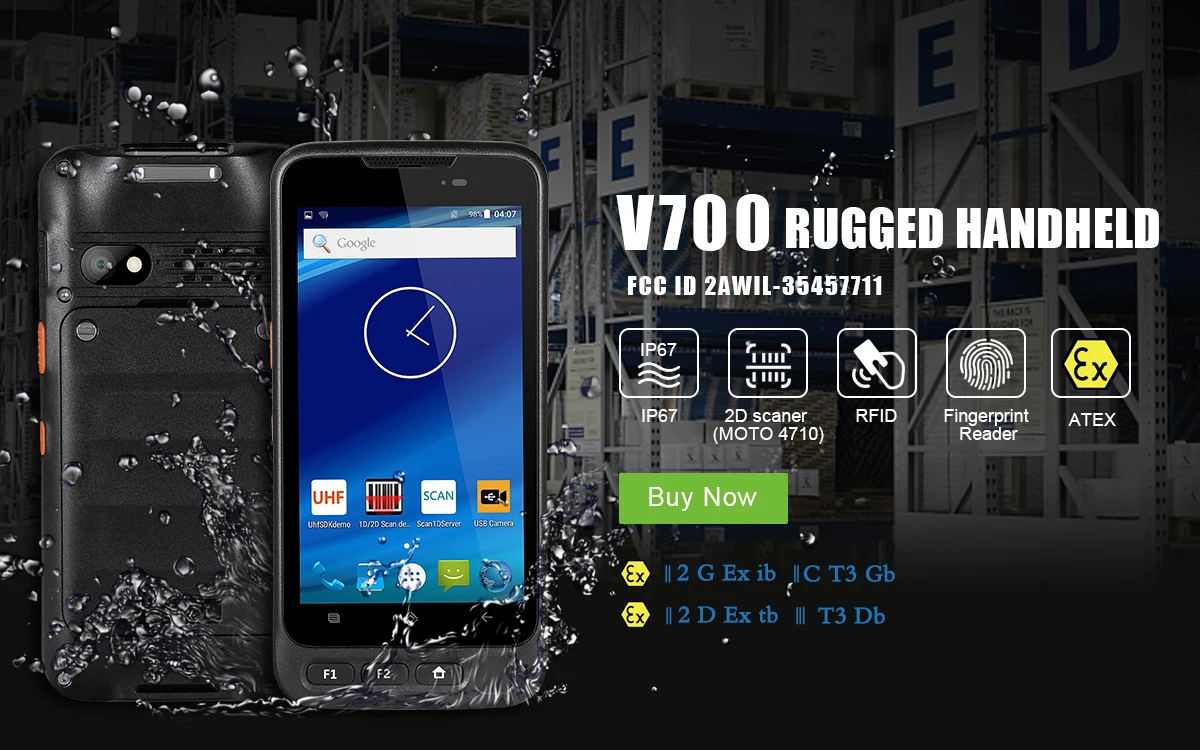This image is categorized under websites but lacks specific indicators of a particular site. The background is predominantly dark with shades of black and gray, depicting what appears to be warehouse shelving. The shelves, made of metal, are labeled with the letters "F.E.E.D.," each letter affixed to a different shelf. Prominently centered on the image in large white text is the model number "B700 Rugged Handheld FCC ID 2AWIL 35457711," followed by features such as "IP67, 2D scanner, Modo 4710, RFID, fingerprint reader, and Atex."

To the left of this text, there are two views of a rugged handheld device, possibly a smartphone, showcasing both its front and back. The phone or its protective case is gray. The screen displays a Google search bar, an analog clock, full battery status, and several app icons, including "UHF Scan Video."